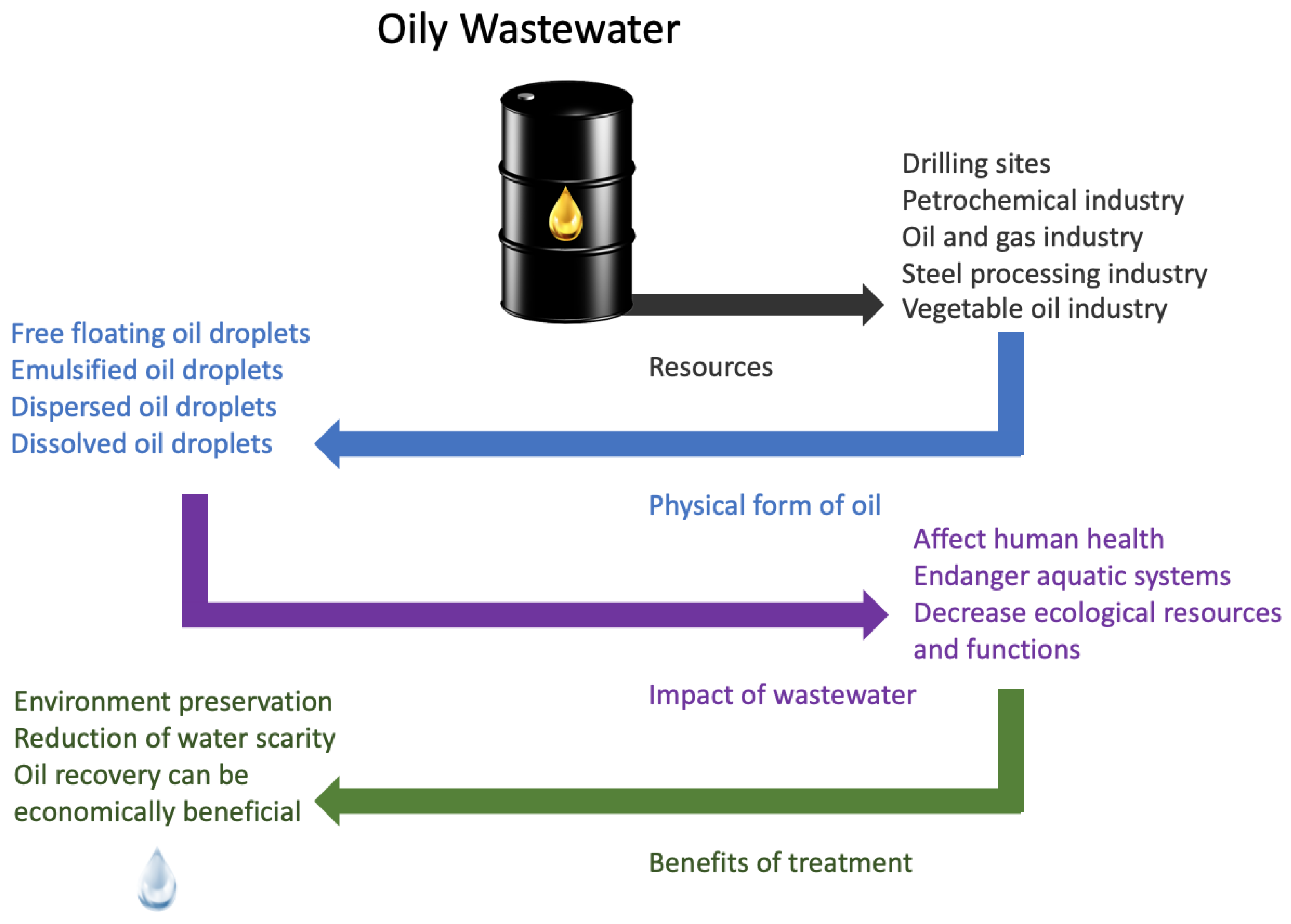This image is a detailed diagram explaining the process and benefits of treating oily wastewater. At the very top, in black lettering, is the title "Oily Wastewater." Below the title is a black drum, symbolizing a barrel, with a flame logo and a golden droplet in its center. A black arrow points right from the base of the drum, leading to text that lists the sources of oily wastewater: drilling sites, petrochemical industry, oil and gas industry, steel processing industry, and vegetable oil industry.

From this list, a blue arrow branches downward to the left, indicating the types of oil droplets present in the wastewater: free-floating oil droplets, emulsified oil droplets, dispersed oil droplets, and dissolved oil droplets. This section represents the physical forms of oil in the wastewater.

A purple arrow emerges downward and right from this section, highlighting the impacts of untreated oily wastewater. It states that these substances affect human health, endanger aquatic systems, and decrease ecological resources and functions.

Following this, a green arrow moves downward and to the left, outlining the benefits of treating oily wastewater. It emphasizes environmental preservation, reduction of water scarcity, and economically beneficial oil recovery. Accompanying this text is an image of a clean water droplet, signifying the outcome of effective treatment. 

The diagram systematically shows the flow from the sources of oily wastewater through its potential hazards to the advantages of proper treatment.